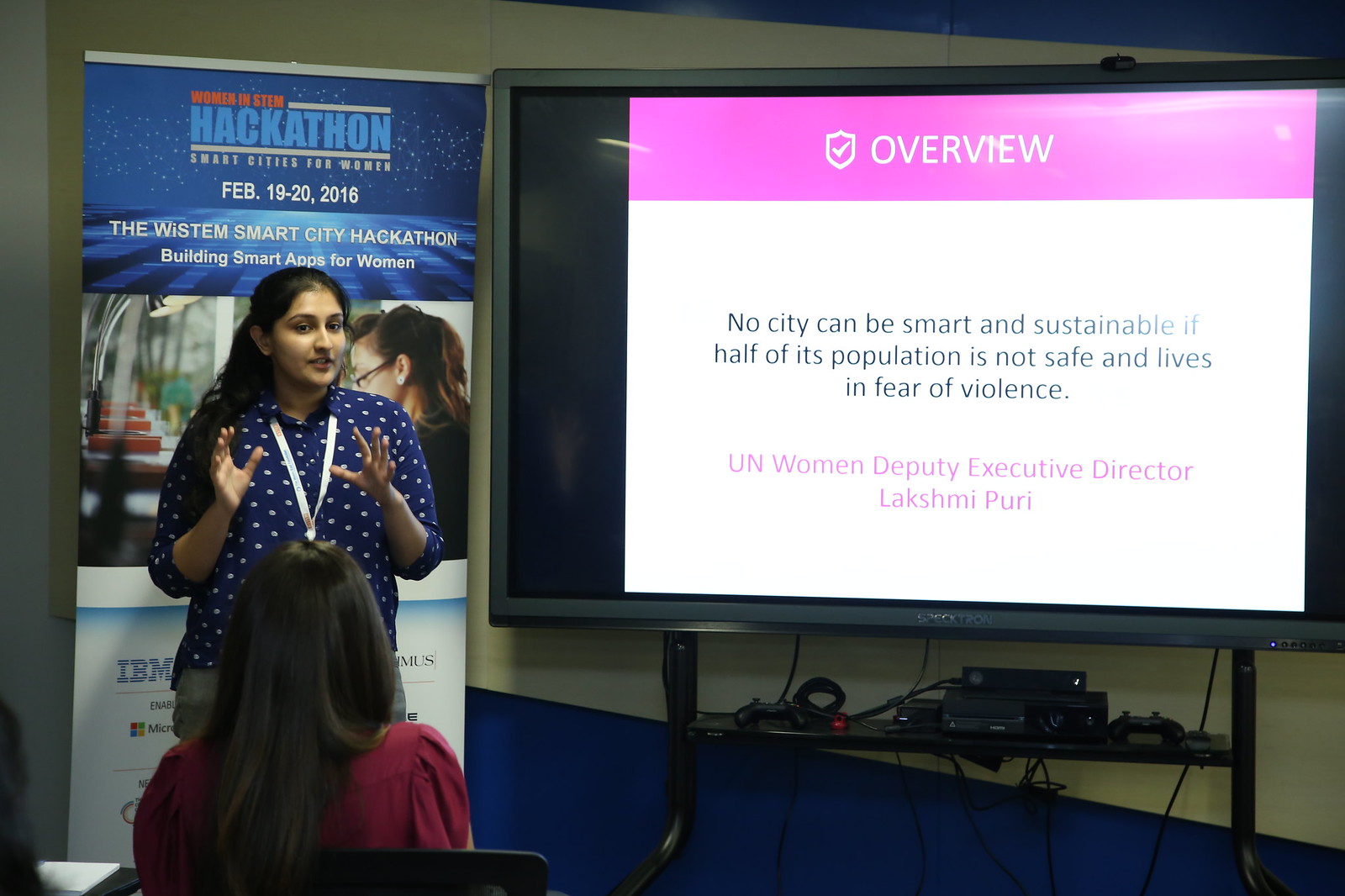In the image, we see an Indian or possibly Arabic woman standing and facing us, gesturing with her hands near her shoulders, and wearing a blue shirt adorned with white dots. Around her neck, she wears a white lanyard, possibly holding a name tag. She appears to be giving a presentation, with a large TV screen to her right. The screen displays a PowerPoint slide with a pink background at the top, where "Overview" is written in white letters. Below, on a white background, black text reads: "No city can be smart and sustainable if half of its population is not safe and lives in fear of violence," and under that, in pink text, it credits "UN Women Deputy Executive Director Lakshmi Puri." Behind the presenter, a sign reads: "Women in STEM, Hackathon, Smart Cities for Women, February 19th through 20th, 2016. The We STEM Smart City Hackathon, Building Smart Apps for Women." In the foreground, below the screen, there is an assortment of black electronic equipment, including what seems to be a controller resembling an Xbox controller and possibly an Xbox itself. To the left side of the image, another woman is seated with her back to the camera, distinguished by her red shirt and long hair cascading past her neck.